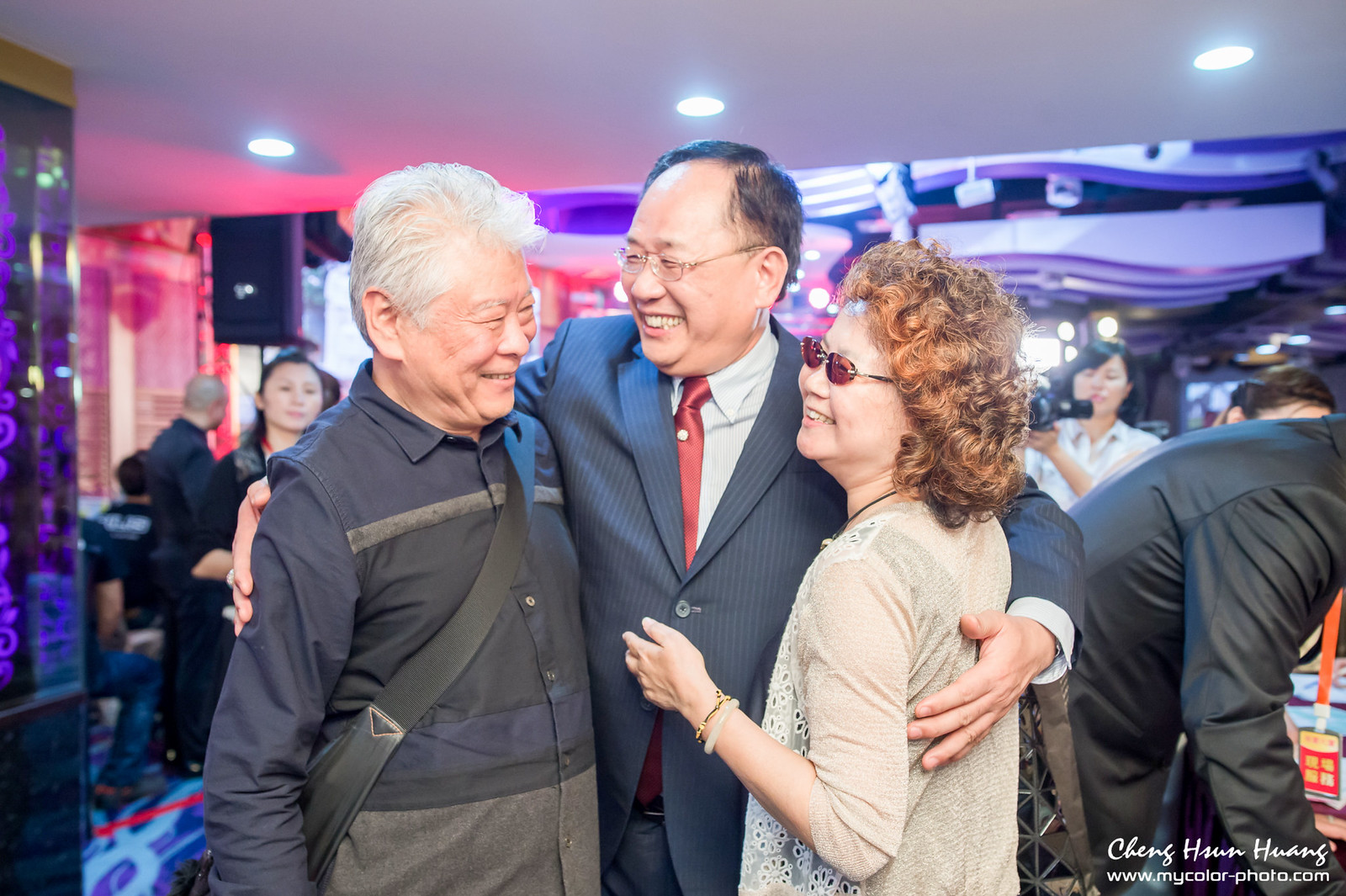In this bright and lively function room with a modern aesthetic featuring recessed pot lights and curved purple decorative panels, the focal point of the rectangular image is three individuals of Asian descent in a warm embrace. The elderly gentleman on the left, with almost completely white hair, is dressed in a dark blue collared shirt and a black strap of a crossbody bag runs across his chest. His smiling gaze is directed towards the woman on the far right. The central figure, a younger man in his 40s, is wearing a pinstripe navy blue suit, a maroon tie, and glasses, and is beaming a broad smile back at the elderly gentleman. His arms are affectionately draped around both the elderly man and the woman on his other side. The woman, with wavy reddish-brown hair, is donning rose-colored sunglasses and a beige blouse, also smiling in the direction of the elderly man. In the background, other attendees in formal attire are slightly out of focus, contributing to the vibrant atmosphere. A camera person is seen recording the event, and various decorative elements, including a speaker and what seems to be keyboard equipment, subtly enhance the scene. The ceiling is white with recessed pot lights, and in the bottom right-hand corner, the name "Chang Haun Huang" and the website "www.mycolorphoto.com" are inscribed, crediting the photographer.